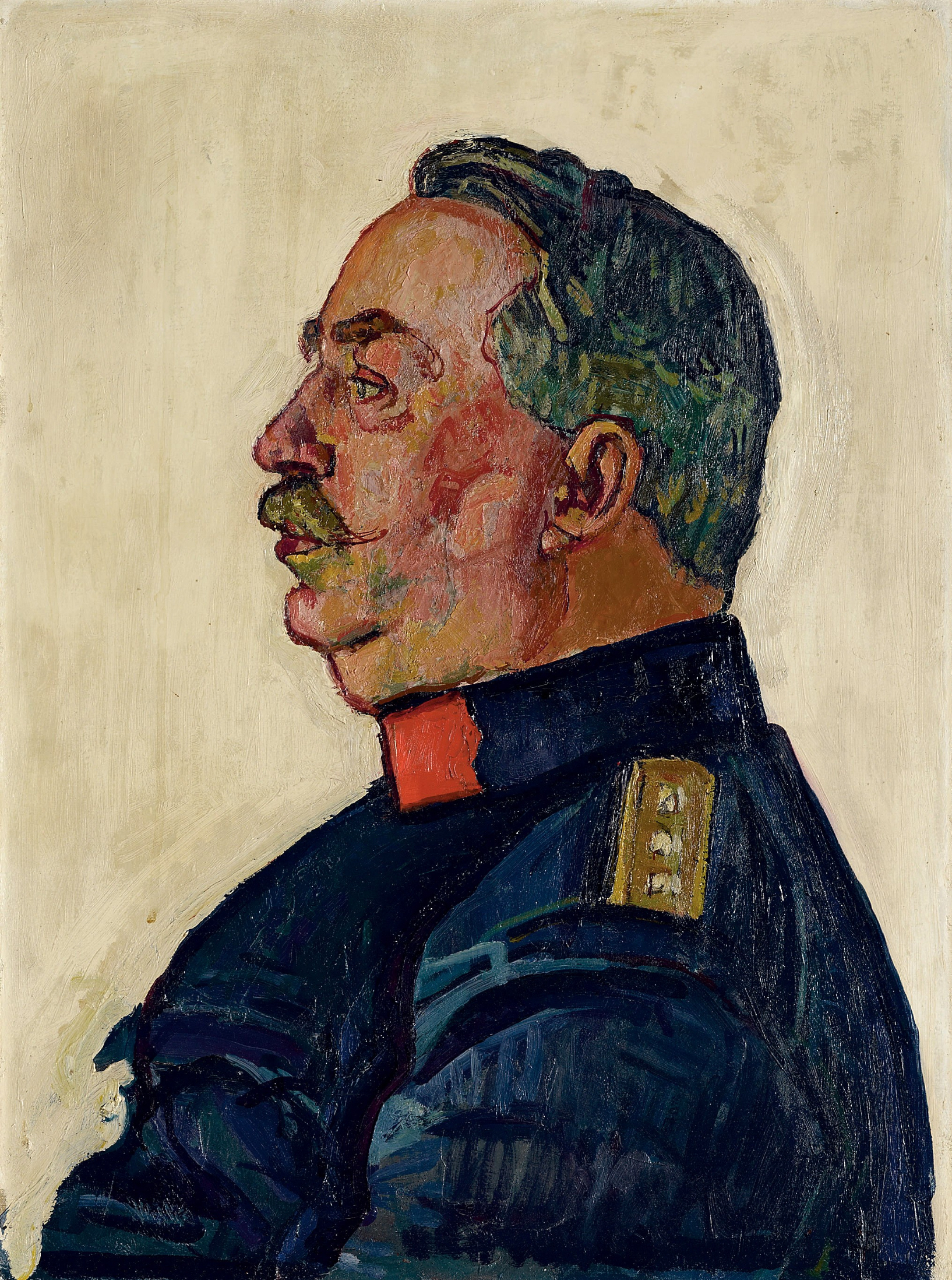This is a watercolor portrait of a man, possibly Joseph Stalin, facing towards the left. His hair is predominantly dark blue with green highlights, slicked back behind his head. His face has a unique color palette, primarily red with hints of orange and amber, complemented by a greenish mustache and a small green patch just below his bottom lip. He appears slightly overweight, with a prominent chin and a double chin underneath it. His eyebrows are brown, and his eyes match the green tones found in his hair and mustache. He is dressed in a blue military uniform, noticeable by the gold-colored bar on the shoulder and a red square at the collar. The background is a mix of ivory, beige, and white with streaks of gray that contour to the man’s head.